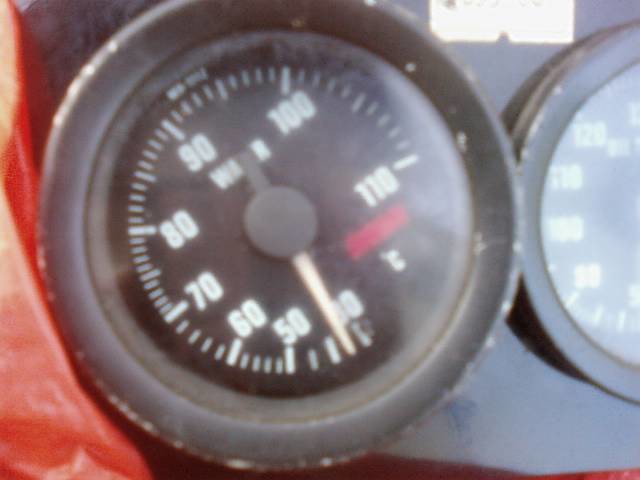This photograph captures a close-up of a vehicle's temperature gauge, likely on a car's dashboard. The image is somewhat blurry and of low quality, which makes the details hard to discern. The gauge has a black face with white markings, indicating temperatures ranging from 40 to 110 degrees Celsius. The numbers 40, 50, 60, 70, 80, 90, 100, and 110 are displayed in ascending order, though the gauge needle obscures some of these markings. The word "WATER" is faintly visible behind the needle, suggesting that this gauge measures the water temperature of the vehicle. A red arc is present above the degree markings, yet its significance is unclear. To the right of the main gauge, half of another gauge is visible, featuring numbers like 90, 100, 110, and 120, but its purpose remains unidentified due to the image's poor clarity. Additionally, a red element is noticeable on the left side of the main gauge, though its function is ambiguous. The entire scene is set against a black background, highlighting the contrasting white and red details.